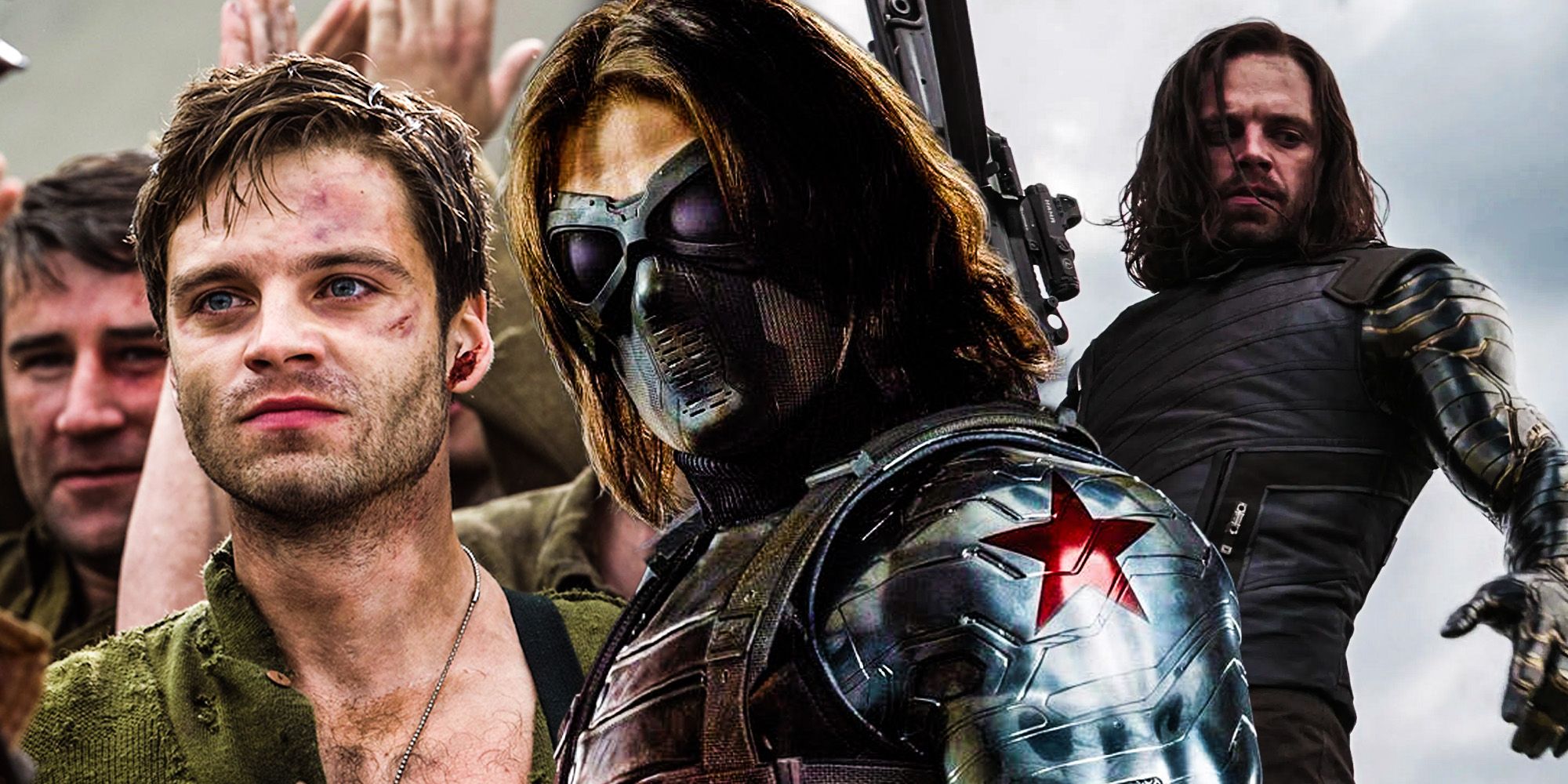In this dramatic scene, a group of four men is captured, potentially from a movie, TV show, or video game, standing against a backdrop of a gray sky. The foreground features a man with long, dark brown hair partially obscured by a mask resembling Darth Vader’s, but allowing his hair to show. The mask, which contributes to his sinister appearance, complements his metallic, military-looking uniform adorned with a red star on his left shoulder. He faces the camera, but his head is turned slightly to the left.

Beside him stands another man, dressed in an olive green army shirt, with short brown hair. He wears dog tags around his neck, signaling a military affiliation, and gazes towards the front left.

Behind the masked man is a figure dressed in dark combat attire, possibly resembling medieval knight gear but anachronistically armed with a semi-automatic weapon. His long brown hair flows freely, adding to the intensity of his warrior-like image.

On the far left, the partially visible face of another man emerges, facing forward. A tan structure and numerous hands, raised as if in celebration or surrender, frame the image to the left, with the scene set under a somber gray sky. The detailed costumes, weapons, and bruised appearances of the men suggest a vivid depiction of conflict, whether it be from a fantastical battle or a gritty, war-torn scenario.